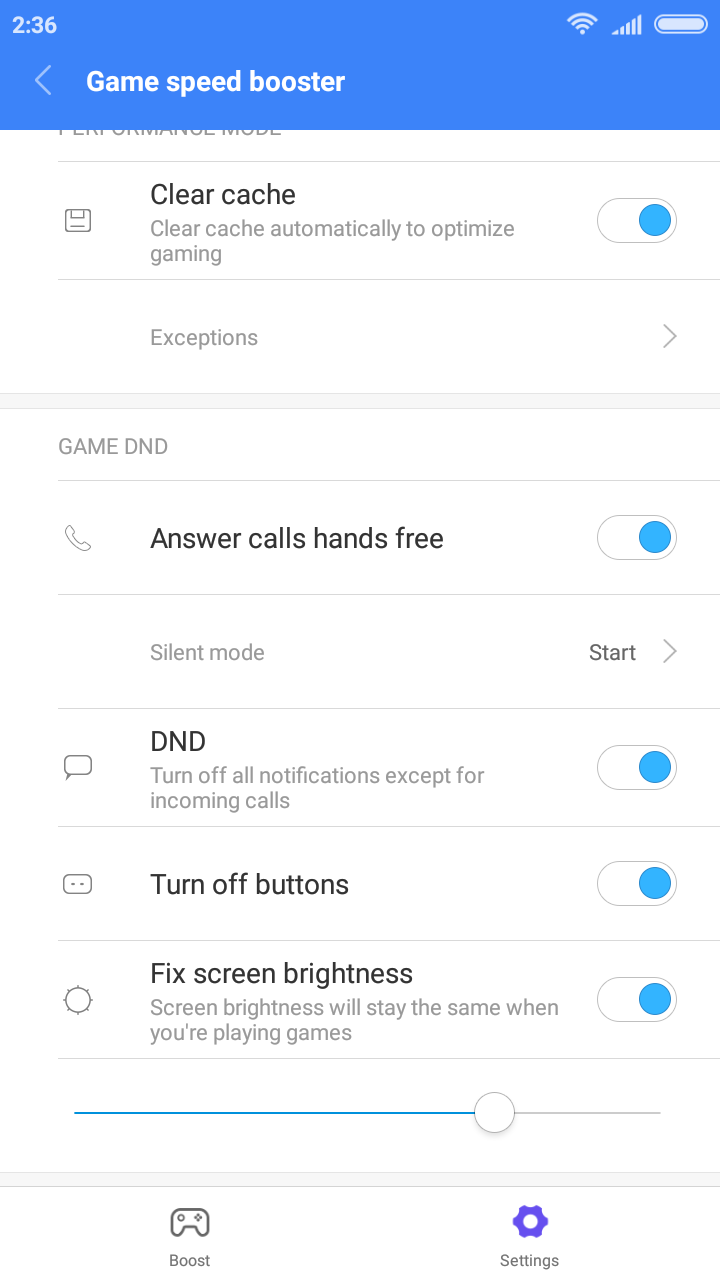**Descriptive Caption:**

Screenshot from an Android smartphone displaying the 'Game Speed Booster' app interface, designed to enhance gaming performance by optimizing various settings. The time shown is 2:36 (unconfirmed if AM or PM). Both Wi-Fi and data connections indicate strong signals, and the battery is nearly full. 

The interface is divided into several sections, each with toggleable options: Clear Cache, Exceptions, Answer Calls, Hands-Free, Silent Mode, Do Not Disturb (DND), Turn Off Buttons, and Fixed Screen Brightness. The Silent Mode option includes a dropdown menu, while Fixed Screen Brightness features a brightness bar at the bottom, ensuring consistent brightness levels during gameplay.